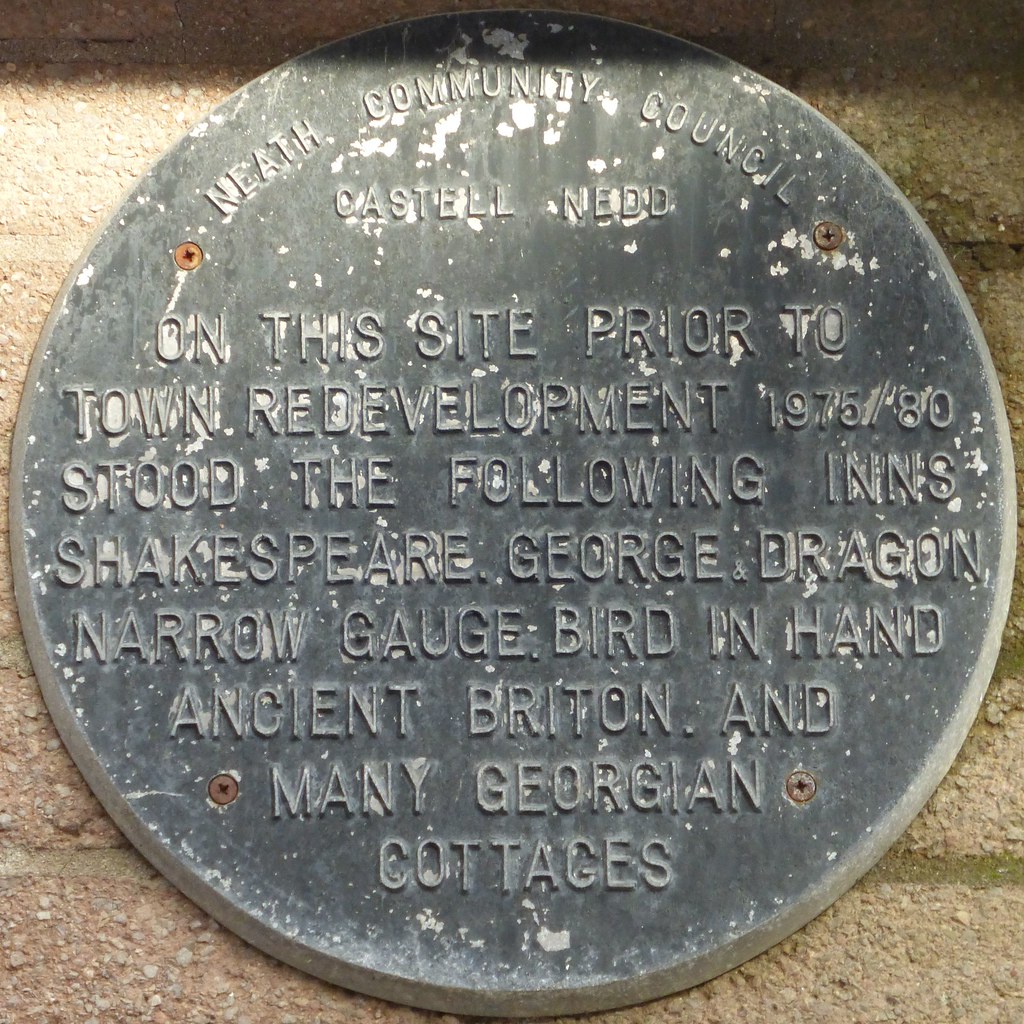The image displays a weathered, round metal plaque, prominently mounted onto a brick wall. The plaque, dark gray with spots of chipping paint revealing white below, is affixed to the wall with four rust-colored screws. The inscription on the plaque reads, "Neath Community Council, Castel Ned. On this site prior to town redevelopment, 1975-80, stood the following inns: Shakespeare, George and Dragon, Narrow Gage, Bird in Hand, Ancient Britain, and many Georgian cottages." The photo is brightly lit, indicating an outdoor setting with ample natural light.